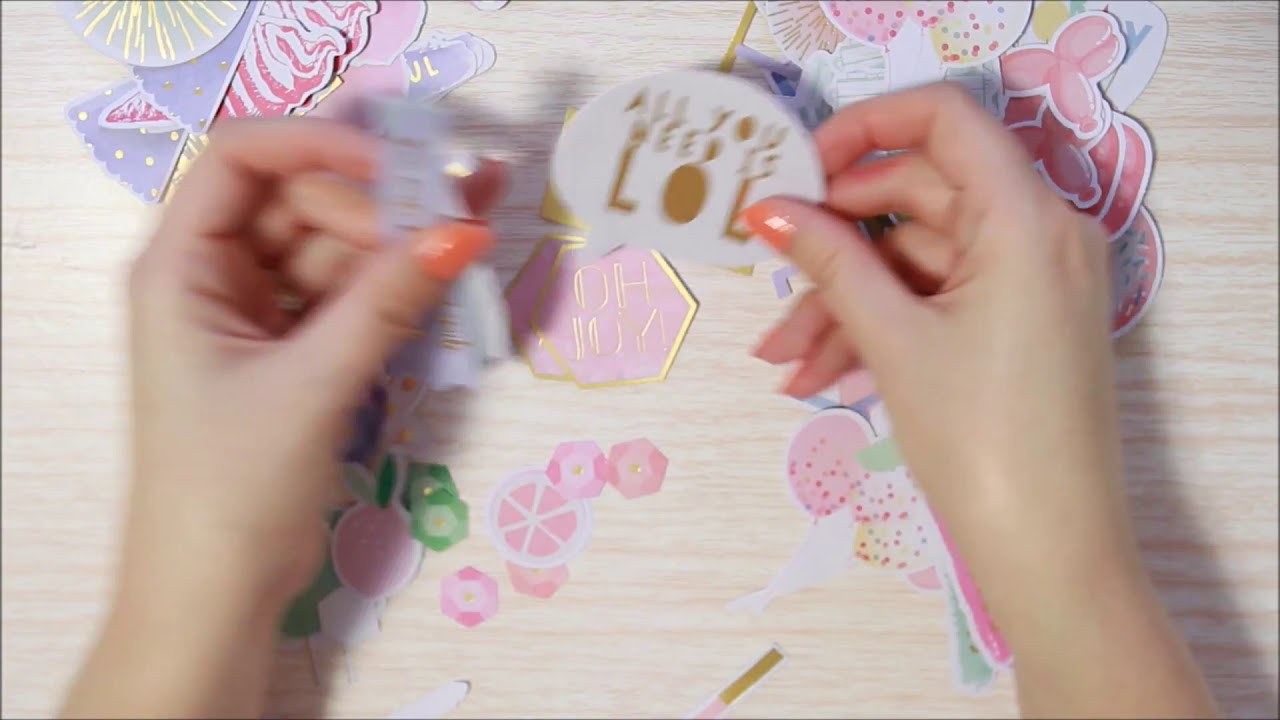In this image, we see a screen capture from a crafting video featuring a fair-skinned woman with peachy-orange nail polish, actively engaged in a creative project on a light wooden table. The table is scattered with various colorful paper crafting components, predominantly in shades of purple, pink, and gold. The woman’s hands, placed prominently in the center of the image, hold different pieces of paper. 

Her left hand, though slightly blurry, holds a purple scrap of paper, while her right hand firmly grasps a white circular piece of paper adorned with the gold-lettered phrase "All you need is LOL." Surrounding her hands, the table is decorated with various paper cutouts, including shapes resembling balloons, balloon animals, orange slices, hexagons, and octagons. Additionally, there are stickers that look like ice cream cones and flowers, suggesting a lively and whimsical crafting project.